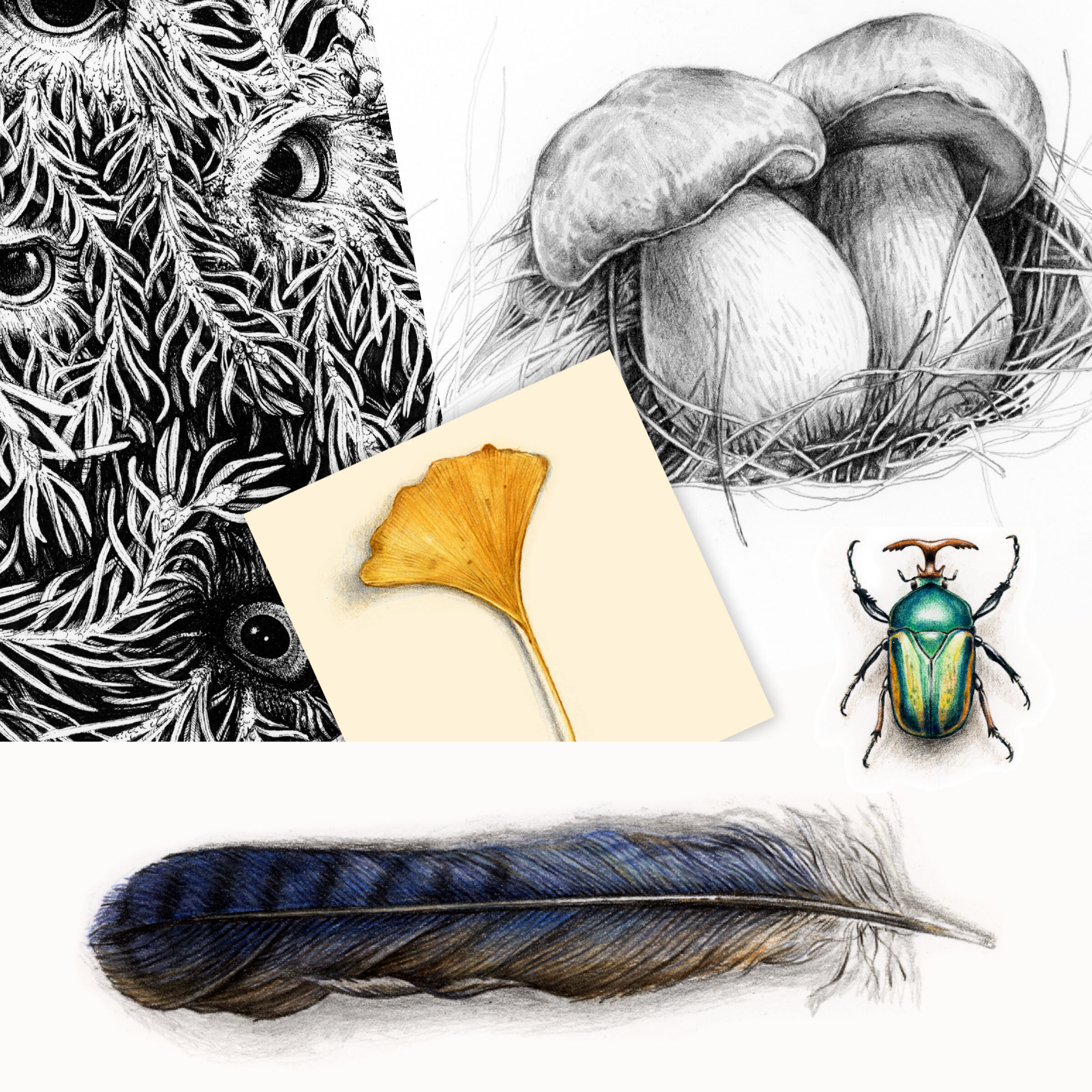The image is a collage composed of five distinct drawings. At the very bottom, a long feather is prominently featured, blending shades of blue and brown. On the right side above the feather, a small, shiny beetle comes into view, showcasing a mix of green and yellow, possibly with a slight blue hue. To the left of the beetle rests a white square containing a striking yellow flower. Behind and partially overlapping these elements, a surreal black-and-white scene emerges, dominated by plant-like forms and four enigmatic, glimmering eyes peering through the foliage. To the top right, the final illustration depicts two large, fully-grown mushrooms in black and white, laying on what appears to be a lightly sketched bird's nest, adding an organic and whimsical touch to the composite artwork.